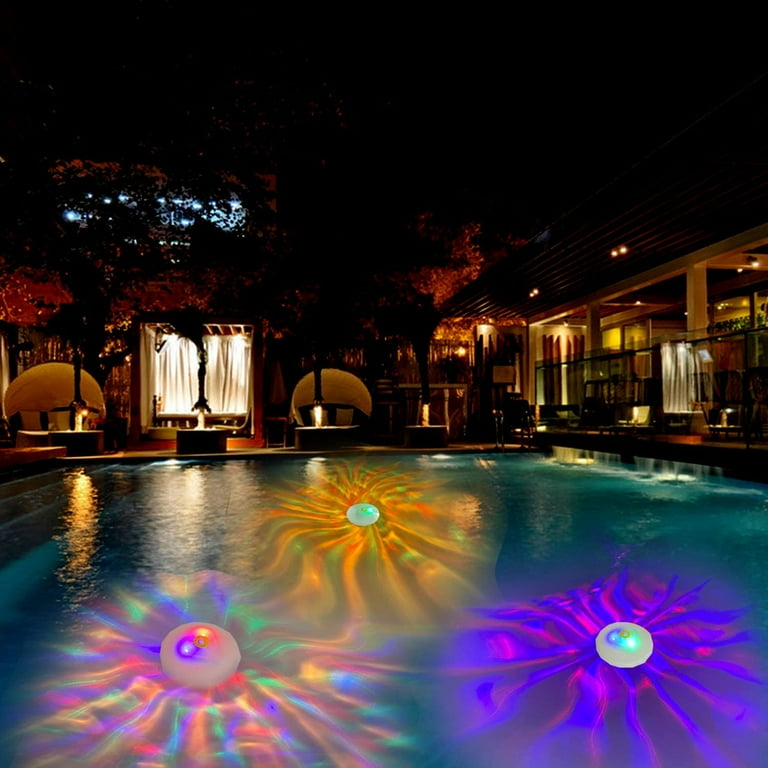In a serene nighttime photograph, a beautifully lit backyard pool takes center stage against a backdrop that is difficult to definitively identify as either a luxurious house, upscale restaurant, or swanky hotel due to the lack of visible occupants and the slightly ambiguous setting. The sky is pitch black, enhancing the contrast and adding to the allure of the scene.

The pool's water shimmers with a light blue texture, accentuated by three luminescent orbs casting a mesmerizing array of LED rainbow colors. The orb on the right glows in purple and red, the one at the top emits hues of yellow and red, and the leftmost sphere dazzles with prismatic rainbow tones, creating an enchanting and almost otherworldly effect in the water.

On the right side of the image, a well-defined porch features a banister with wooden pillars and a glass-like fence, allowing diffused light to pass through. Adjacent to the pool are two semi-circle couches and two coffee tables, arranged in a cozy, dimly lit lounge area. Between these couches stands a wooden booth adorned with a white curtain. Red-tinted foliage from nearby trees adds a pop of color to the otherwise tranquil scene. 

In front of the seating, four cylindrical tree pots hold four trees that contribute to the natural yet manicured aesthetic of the backyard. The entire area radiates exclusivity and elegance, showcased distinctly against the dark night sky.